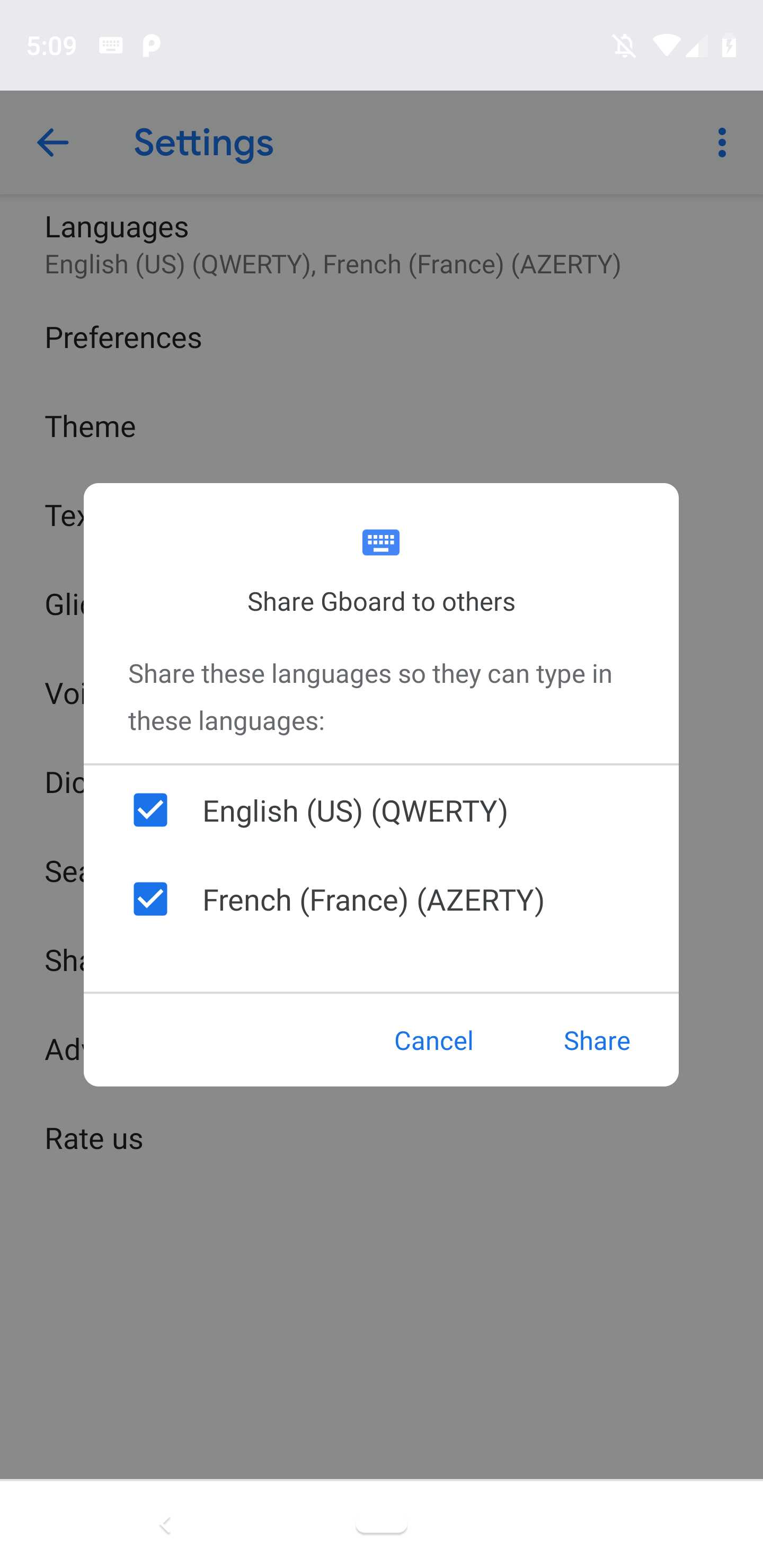The image is a screenshot taken from a mobile phone displaying the Gboard app's settings menu. The top bar is a light gray, housing several status indicators. On the upper left-hand corner, the time is displayed as 5:09. Adjacent to it is a white square icon, followed by a white "P" icon. Moving to the far right, there are additional icons: a white bell with a line through it indicating the ringer is silenced, the Wi-Fi signal icon, cellular signal bars (two out of four filled), and a white battery icon.

Below this top bar, the main content of the screenshot is predominantly black and white. Over this, a white message box prominently stands out. The message box contains a blue keyboard graphic at its center and text instructions in black: "Share Gboard to Others." Following that, in gray text, it states: "Share these languages so they can type in these languages."

Further below, there are two blue selection boxes with white checkmarks. The first box reads, "English (US) QWERTY," with "QWERTY" in all caps. The second box reads, "French (France) AZERTY," with "AZERTY" also in all caps. Beneath these options, there are two clickable blue text options: "Cancel" and "Share."

In the gray, blurred background, the underlying Settings menu is visible, featuring a list of options. The heading is "Languages," listing "English (US) QWERTY" and "French (France) AZERTY." Below those, the menu options include "Preferences," "Theme," and "Text." The subsequent options are partially cut off, showing only fragments of text: "GLI," "VO," "DI," "SE," "SH," "AD," and "RATE US." On the far left of the menu is a back arrow, and on the far right are three vertical dots, indicating additional options.